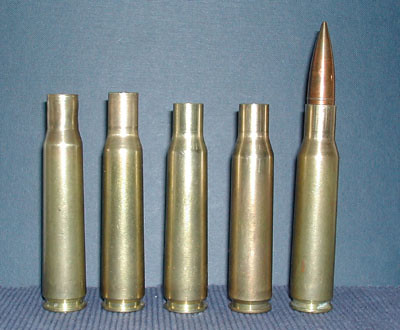The photograph features five bullet casings, each standing upright against a textured surface that appears to be gray with a hint of blue, resembling fabric. The background is a medium gray-blue, possibly concrete. The casings themselves are brass or gold in color, with the first four being empty shells and the last one on the right containing a pointed, inch-long copper bullet. The two casings on the far left are slightly taller than the two adjacent to them, while the final casing with the bullet matches the height of the shorter pair. No people or text are present in the image. The setting and arrangement draw attention to the astonishing sharpness and potential lethality of the lone copper-tipped bullet among the otherwise hollow shells.